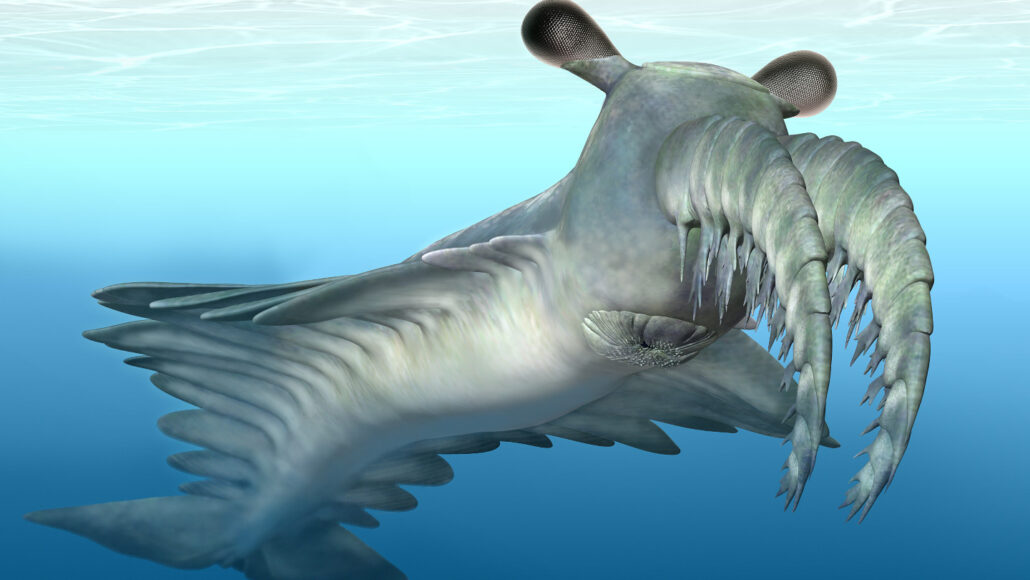This highly detailed 3D rendering showcases a fantasy prehistoric underwater creature in a rectangular image set within a vast, blue ocean. The top half of the picture features a lighter blue, indicating proximity to the white, sunlit surface, while the deeper regions transition to a darker blue. Positioned centrally, the creature exhibits similarities to a shark in texture and coloration, with a gray back and a white underside. Distinctive features include multiple thick, gray tendrils along its sides and two large, segmented, shrimp-like tendrils extending from the front of its mouth. The head houses a circular mouth on the underside, and two eyestalks topped with large, bulbous black eyes protrude from the top. Its flat, dual-triangular tail fin contrasts with the bizarre complexity of its form, highlighting this creature as a product of imaginative artistry rather than reality.